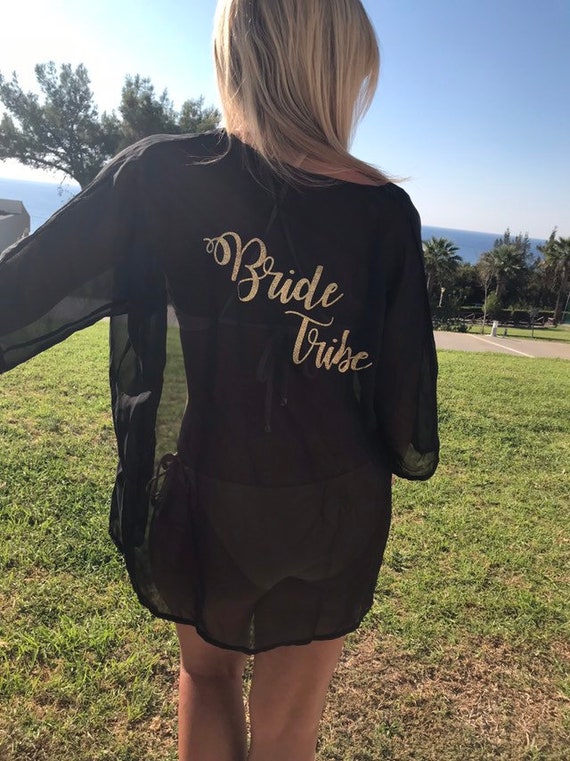The photograph captures the back of a young woman in a colorful, sunny outdoor setting, likely a park. She is wearing a sheer, long-sleeved black top with gold cursive lettering that reads "Bride Tribe." Underneath her top, she appears to be wearing a light-colored bikini, visible through the transparent fabric. The woman has long, straight blonde hair and a light complexion. She walks across a grassy area, which is mostly green but shows some browning patches. The scene includes a tennis court or some asphalt area in the background, accompanied by trees and possibly palm trees. The sky above is a brilliant blue, enhanced by white puffs of clouds, emphasizing the bright and clear day.